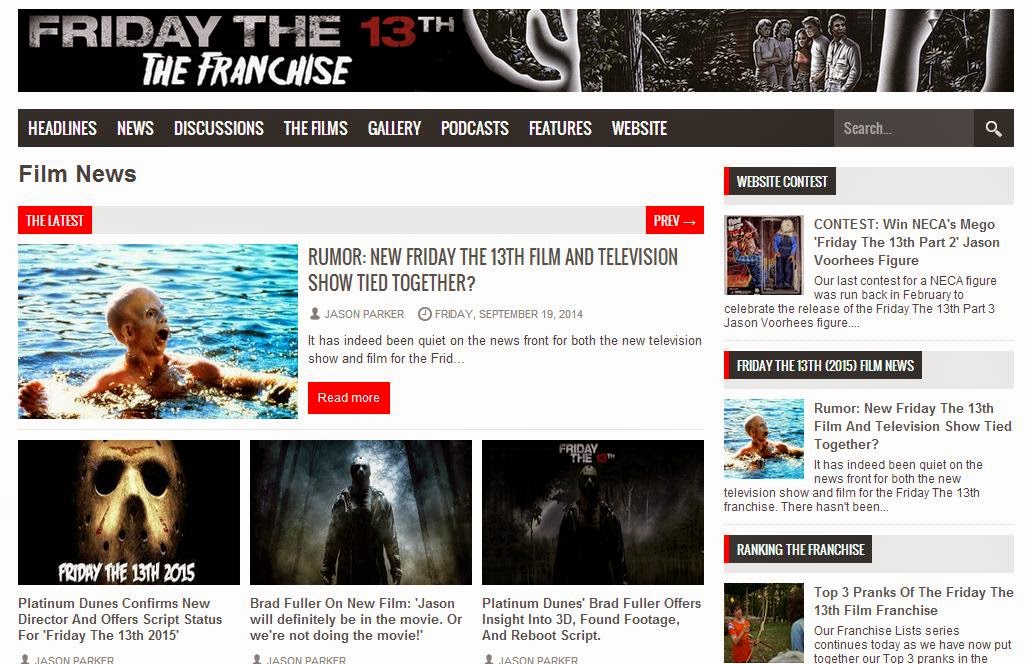This is a detailed caption for an image depicting a cropped screenshot of the "Friday the 13th: The Franchise" webpage.

---

The cropped screenshot showcases the "Friday the 13th: The Franchise" webpage. At the top of the page, there is a large header featuring the title "Friday the 13th: The Franchise" in a mix of fonts and colors: "The Franchise" is in a very large white font, "Friday the 13th" in light gray, and the number "13" highlighted in red. To the right side of the header, there is a group photo of the film's cast.

Beneath the header is a navigational bar with several categories, including "Headlines," "News," "Discussions," "The Films," "Gallery," "Podcasts," "Features," and "Website." To the far right of this bar is a search bar.

Further down, the body of the webpage is set against a white background. On the top left in large gray letters is the section title "Film News," with a red box below it labeled "Latest." Next to it is a thumbnail with the headline "Rumor: New Friday the 13th Film and Television Show Tied Together" beside it. Below this headline, the author's name and date of publication are shown, followed by a red "Read More" box.

Towards the bottom of the screenshot, three additional thumbnails are displayed, each accompanied by a story headline and the author's name at the bottom. On the right, three vertical listings are visible, including "Website Contest," "Friday the 13th Film News," and "Ranking the Franchise."

The remaining content of the webpage is cropped out in the screenshot.